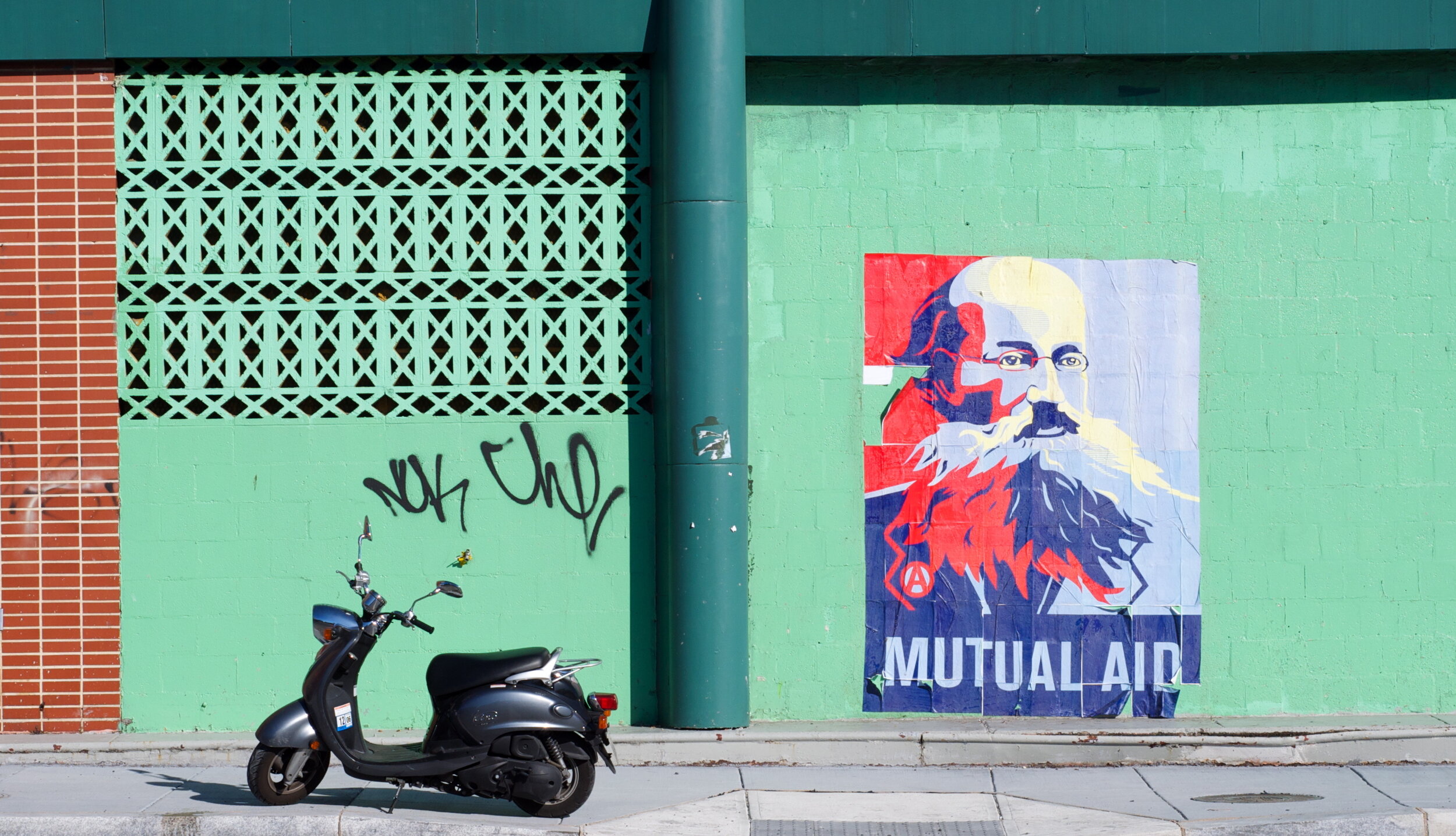The image showcases an outdoor wall, depicted in a horizontal rectangular format. The wall is predominantly green, with a dark green pillar at its center. On the left side of the pillar, the wall exhibits a red brick section comprising three rows of bricks transitioning into a light mint green wall featuring a lattice pattern on the upper portion adorned with black graffiti. Although the graffiti is not fully legible, it provides an artistic element to the scene. Parked in front of this green wall is a dark motor scooter. To the right of the pillar, the green wall extends further, where a poster prominently displays the image of a bald man with glasses, a long beard, and a red, white, and blue mustache, with the words "Mutual Aid" inscribed. The scooter rests on a light gray, slightly bumpy, tiled sidewalk, adding to the urban atmosphere of the image.